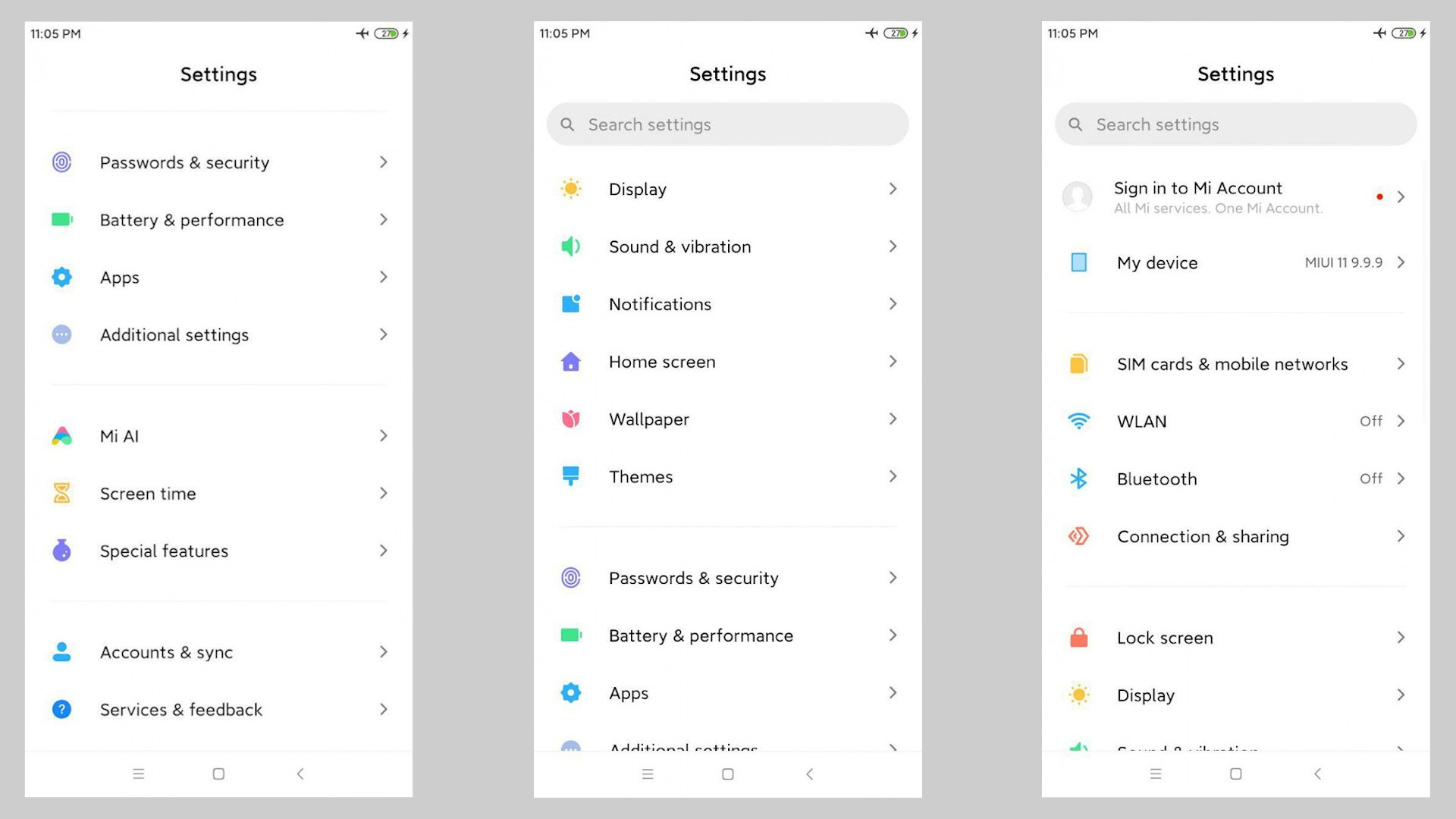Here is the revised and detailed caption for the image:

"The image consists of three separate smartphone screenshots, each displaying the 'Settings' menu with a gray background. The current time is 11:05 p.m., and airplane mode is activated on all three screenshots.

In the first screenshot, the following options are visible: 'Passwords and Security,' 'Battery and Performance,' 'Apps,' 'Additional Settings,' 'MIAL' (note the lowercase 'i' and 'l'), 'Screen Time,' 'Special Features,' 'Accounts and Sync,' and 'Services and Feedback.'

The second screenshot shows a slightly different arrangement with these options listed: a search bar at the top, followed by 'Display,' 'Sound and Vibration,' 'Notifications,' 'Home Screen,' 'Wallpaper,' 'Themes,' 'Password and Security,' 'Battery and Performance,' 'Apps,' and 'Additional Settings.'

The third screenshot also starts with a search bar and includes: 'Sign in to my MI Account,' 'My Device,' 'SIM Cards and Mobile Networks,' 'WLAN' (in all capital letters, which is turned off), 'Bluetooth' (which is off), 'Connection and Sharing,' 'Lock Screen,' and 'Display.'"